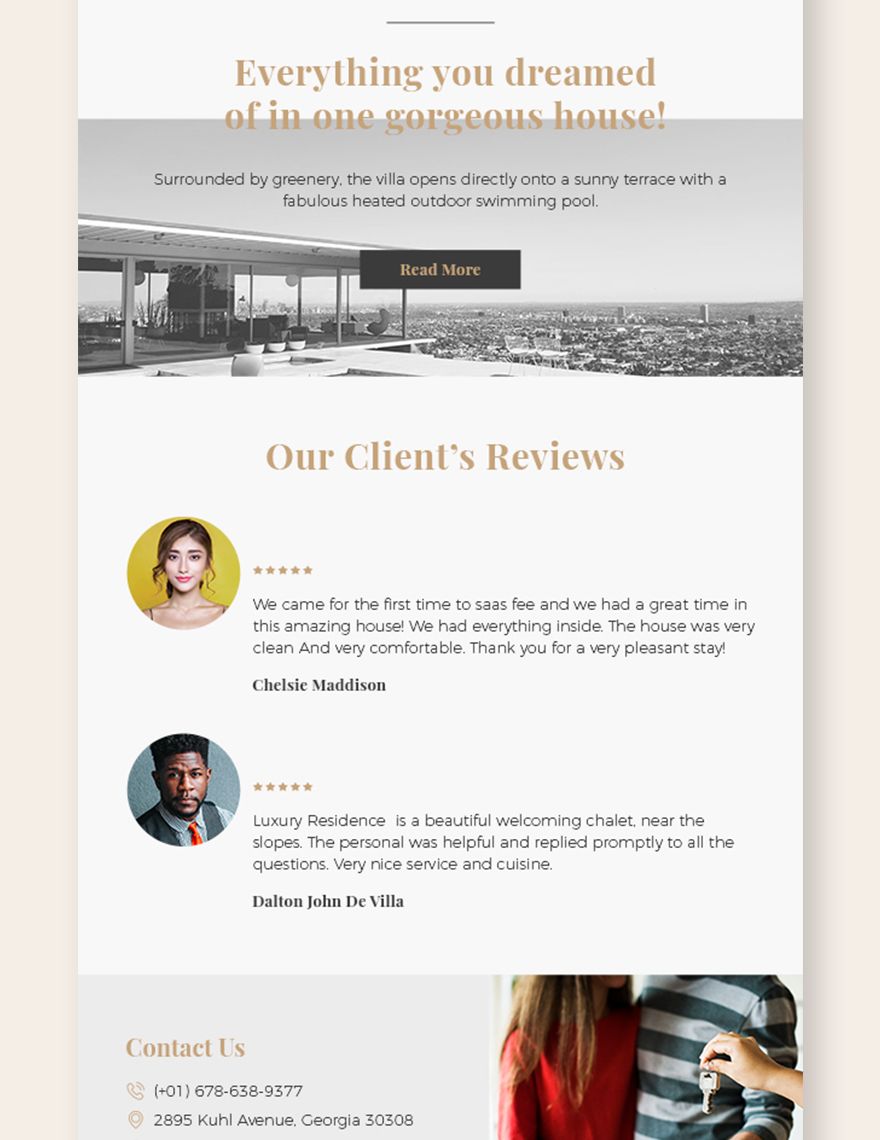The image showcases a stunning villa that epitomizes luxury and comfort. The villa boasts an inviting sunny terrace, seamlessly connected to a fabulous, heated outdoor swimming pool. The scenic view is complemented by lush greenery that encapsulates the dream home ambiance. 

Above the image, a brown text banner entices you with a message: "Everything you dreamed of in one gorgeous house." To the right, a black bar with the call to action "Read More" hints at further details about this exquisite property.

In the foreground, there is a personal testimonial section with a yellow background displaying 5 gold stars. One testimonial, authored by Chelsea Madison, reads: "We came for the first time to SASV. We had a great time in this amazing house. We had everything inside. The house was very clean and very comfortable. Thank you for a very pleasant day." The consistent 5-star rating emphasizes the high satisfaction of visitors.

A secondary testimonial from Dalton John Devia praises the property for its strategic location and exceptional services: "It's a beautiful, welcoming chalet near the slopes. The person was helpful in replying promptly to all the questions. Very nice service and cuisine." This testimonial also features a 5-star rating.

On the left side of the image, contact details are prominently displayed: "Contact Us: +01678-638-9377, 2895 Cole Avenue, Georgia 30308." The visual elements include a person in a red shirt and another individual holding up a set of keys, signifying the seamless and personal service provided to clientele.

Overall, this detailed caption paints a vivid picture of an idyllic property perfectly suited for a luxurious and relaxing stay.